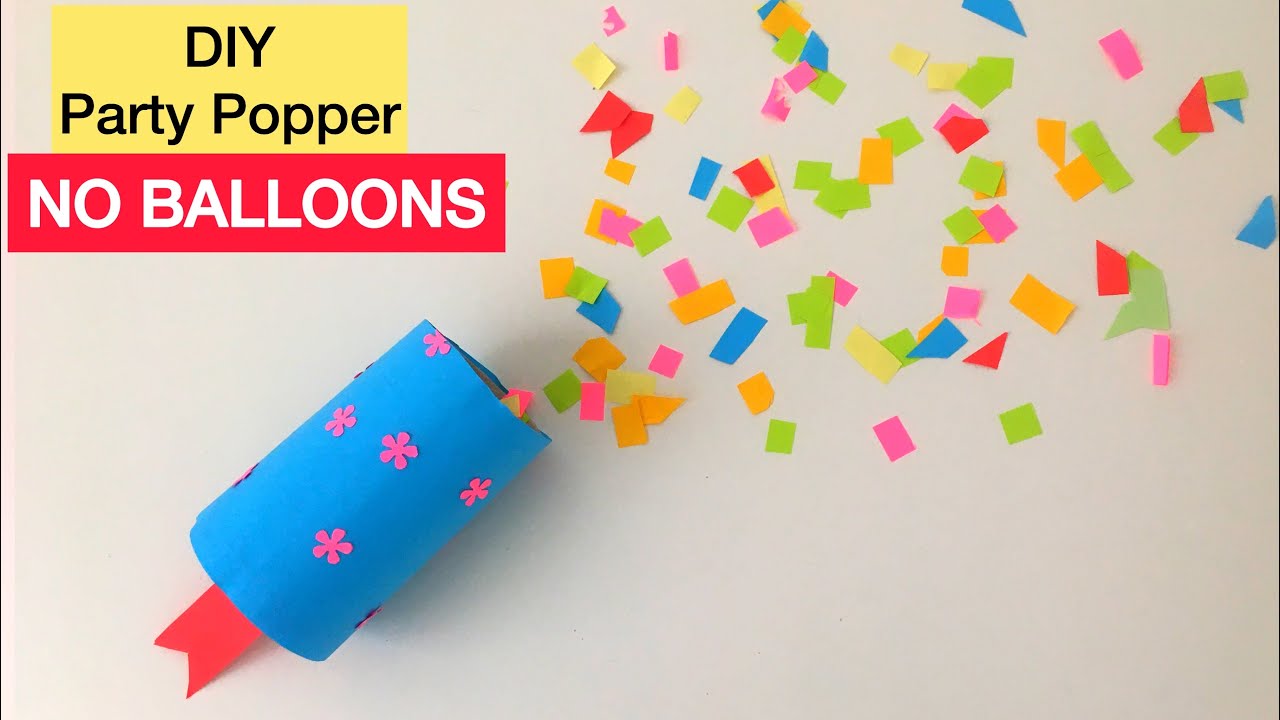This is a color image showcasing a DIY (do-it-yourself) party popper. The scene is set against an off-white background, with a yellow square in the top left corner featuring bold black text that reads "DIY Party Popper," and a red rectangle beneath it with white text stating "No Balloons." The focal point is a blue cylindrical party popper positioned diagonally in the bottom left corner, pointing up towards the top right. The popper is decorated with pink paper flowers and has a red ribbon tail at the bottom end. Decorative paper pieces in orange, green, blue, pink, yellow, and purple are depicted as if they are bursting out of the popper, although they all lie flat on the surface, giving an artsy and visually appealing impression of confetti explosion. This entire display is crafted from cut-out paper, emphasizing a handcrafted, artistic representation of a typical party popper.